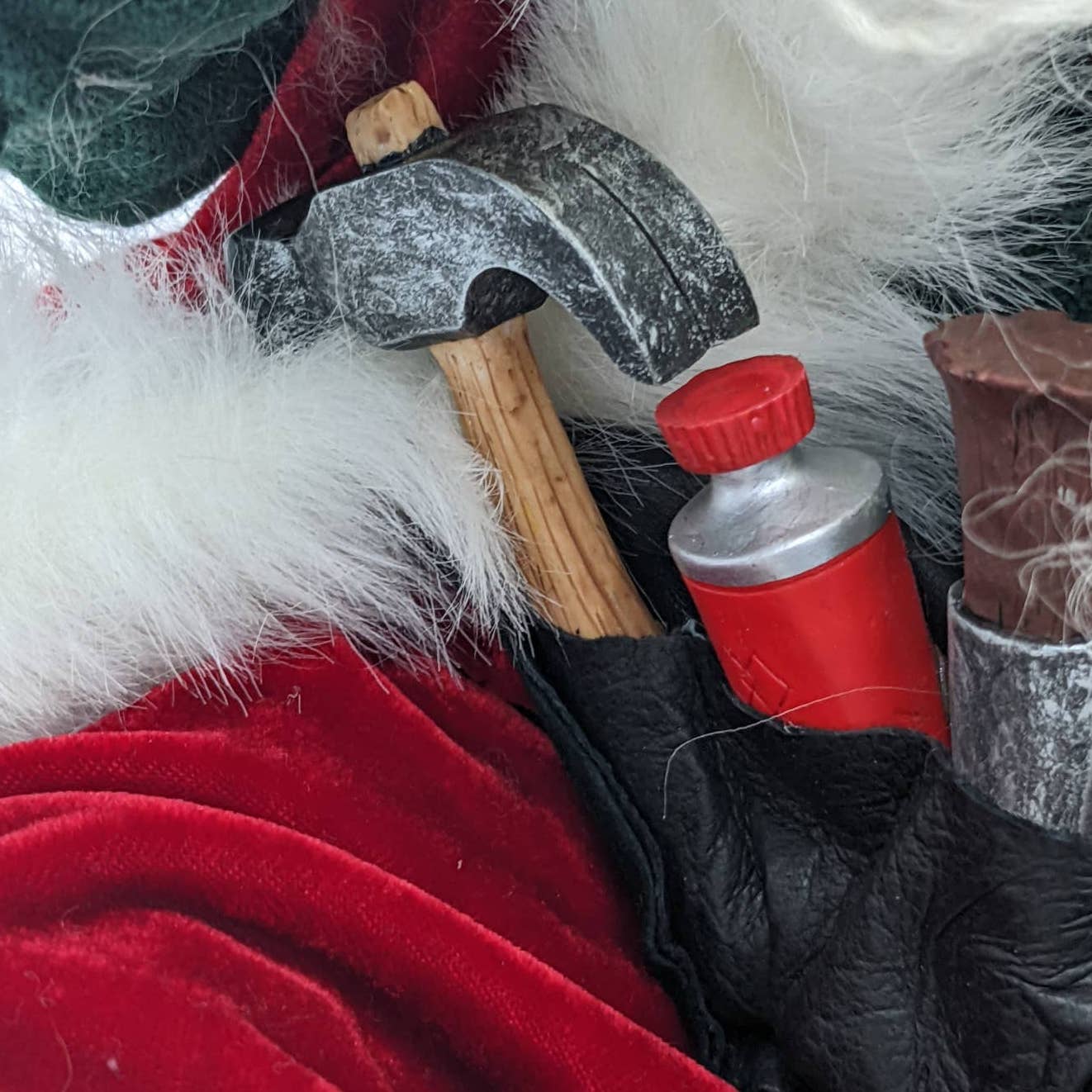This close-up image showcases a variety of tools set against a festive backdrop resembling a Santa Claus outfit. The background is predominantly a red velvet material, accented with white, synthetic fur trim, evoking the look of Santa's suit. Within the scene, a few tools are strategically placed, drawing attention to a black leather tool belt holder positioned towards the lower right corner of the image. Resting in the left pocket of this holder is a distinctive hammer with a wooden handle and a silver or black head. The middle pocket contains a red and silver tube with a red cap, possibly a glue tube, while the third pocket holds a brown and silver item, potentially another tool post. There is also a hint of green material in the upper left corner, perhaps a tablecloth, enhancing the rich contrast of colors and textures, including velvet, fur, leather, metal, and plastic. Overall, the image suggests a blend of holiday cheer and practical utility.